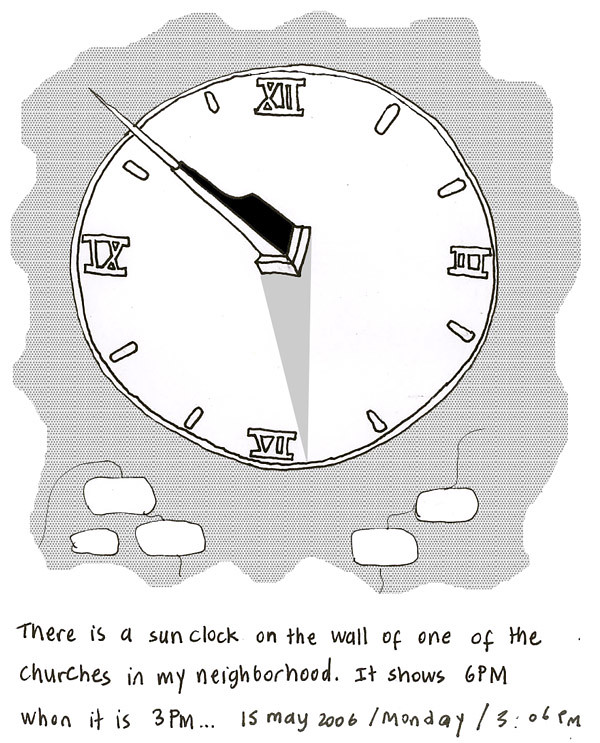This digital illustration depicts a sun clock, or sundial, set against a white background with a wavy, circular gray inner border resembling a crisscross pattern. The sundial, crudely drawn in a hand-drawn style with a black pen outline, displays Roman numerals at the 12, 3, 6, and 9 o'clock positions, while notches mark the other hours. The central gnomon, resembling a skyscraper's spire, casts a shadow indicating the time. Below the illustration, in digitally handwritten text, it reads: "There is a sun clock on the wall of one of the churches in my neighborhood. It shows 6pm when it is 3pm... 15 May 2006 / Monday / 3:06pm." The text, with a spelling mistake ("whon" instead of "when"), suggests it might have been written by a child or someone learning English, hinting that this illustration could be part of an educational project or digital learning activity.